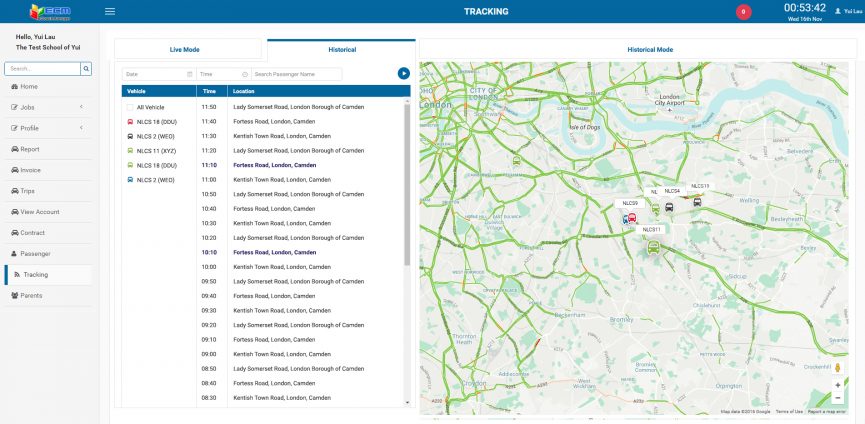The top left corner of the image prominently displays the letters "EGM" along with an icon resembling a hamburger menu. The interface features a primary color scheme of blue with red elements for highlights and tracking indicators. A prominent red circle features the number "005342". Next to it is a greeting that reads "Hello, Yui Lau," followed by the identifier "The Test School of Yui".

The interface contains numerous function tabs including "Search", "Elementary Life", "Home", "Jobs", "Profile", "Report", "Invoice", "Trips", "Fuel Count", "Contract", "Passenger", "Tracking", "Parent", "Life Mode", "Historical", and "Historical Mode". Below these tabs, there are options for "Date" and "Time" filters, as well as a search bar for inputting a passenger name or vehicle ID.

In the section for tracking vehicles, several vehicle identifiers such as "NLCS18", "NLCS2", "WG", "NLCS11", "KXYZ", "NLCS18DOU", "NLCS2" are listed alongside timestamps including "11:50", "11:40", "11:30", "11:20", "11:10", "10:50", "10:40", "10:30", "10:20", "10:10", and additional times noted as "94930", "92910", "9850", "9840", and "9830".

Locations such as "IE Summerset Fortress Road, London, Camden" appear frequently in the list, with the address "Fortress Road, London, Camden" showing up consistently across different timestamps like "11:10" and "10:10".